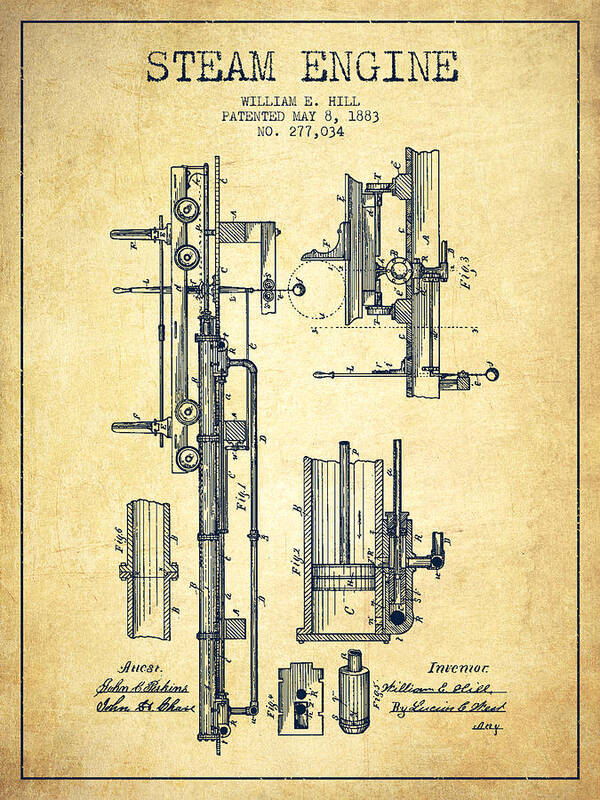The image depicts an aged, yellowed piece of parchment paper, approximately one and a half times taller than it is wide, suggesting a portrait orientation. The paper bears the title "Steam Engine" at the top in large black capital letters, followed by the name "William E. Hill" and the text "Patented May 8, 1883, Number 277,034" in smaller, centered text. 

Below the header, the majority of the document is occupied by intricate black-and-white technical drawings of the steam engine, illustrating various parts and their configurations. The drawings are meticulously labeled with call-outs and letters, presumably corresponding to detailed descriptions or parts lists on a separate page.

At the bottom of the document, the text "Inventor" appears, followed by William E. Hill's signature. On the opposite side, there are additional signatures—possibly witnesses to the patent—with one legible as "Lucere" and others less decipherable, potentially including names like John B. something.

The entire document is framed by a thin black border, enhancing its formal and vintage appearance. Additional handwritten notes in small script decorate the sides, adding to the historical and technical depth of the artifact.